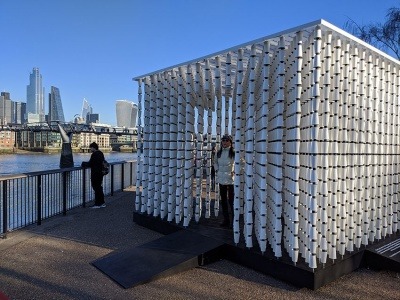The photograph is a vibrant, photorealistic capture of a bustling city riverwalk. In the foreground, a broad concrete promenade stretches out alongside the river, which is bordered by a sleek metal guardrail. On the left side of the image, the glimmering river extends into the distance, where a bridge gracefully arches over the water. Beyond the bridge, the impressive city skyline is visible, featuring several distinctive skyscrapers, including a tall black wedge-shaped building, a step-like structure reminiscent of the Empire State Building, and a vase-shaped tower.

Central to the scene is a striking contemporary art installation on a black, square platform, which appears to be constructed from painted wood. The installation includes what looks like vertical poles adorned with segmented white pieces, possibly styrofoam cups or sections of PVC pipe, creating a visually intriguing, open framework. A black ramp leads up to the installation, allowing access from multiple sides. A woman, wearing a white sweater, long black hair, sunglasses, and a cap, stands inside the structure, seemingly posing for a photograph.

In the background, a man stands by the guardrail, gazing out over the serene river, adding a human element to the tranquil yet dynamic urban setting. The bright blue sky overhead enhances the overall sense of daytime vitality in this snapshot of modern city life.